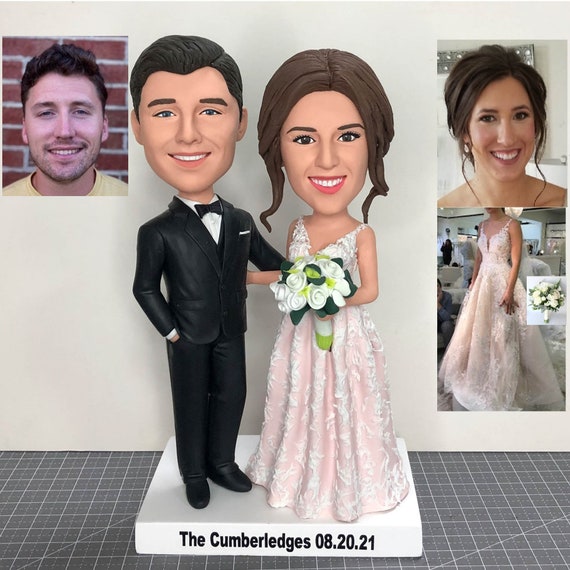This detailed image showcases a custom wedding cake topper featuring bobblehead renditions of a bride and groom, identified as "The Cumberledges," commemorating their wedding date of 08.20.21. Positioned on a white square base with raised edges, the base bears an inscription in black print: "The Cumberledges 08.20.21." The groom is on the left in a black tuxedo with a white shirt and black bow tie. His right hand rests casually in his pocket while his left hand extends behind the bride's waist. He has short dark brown hair, brown eyebrows, and a smiling expression. The bride stands to his right, adorned in a sleeveless, v-neck wedding dress with a pink hue and white lace overlay. She holds a bouquet of white calla lilies, wrapped in a white ribbon. Her hair is styled in an elegant updo with some curls framing her face.

Above the figures, on the left side, there is a small portrait photograph of the groom dressed in a yellow shirt, set against a brick wall. On the right side is a corresponding small portrait photograph of the bride, showing her with her wedding dress and bouquet in a ballroom setting. This juxtaposition highlights the striking resemblance between the lifelike dolls and their real-life counterparts, making it a perfect keepsake for their special day.